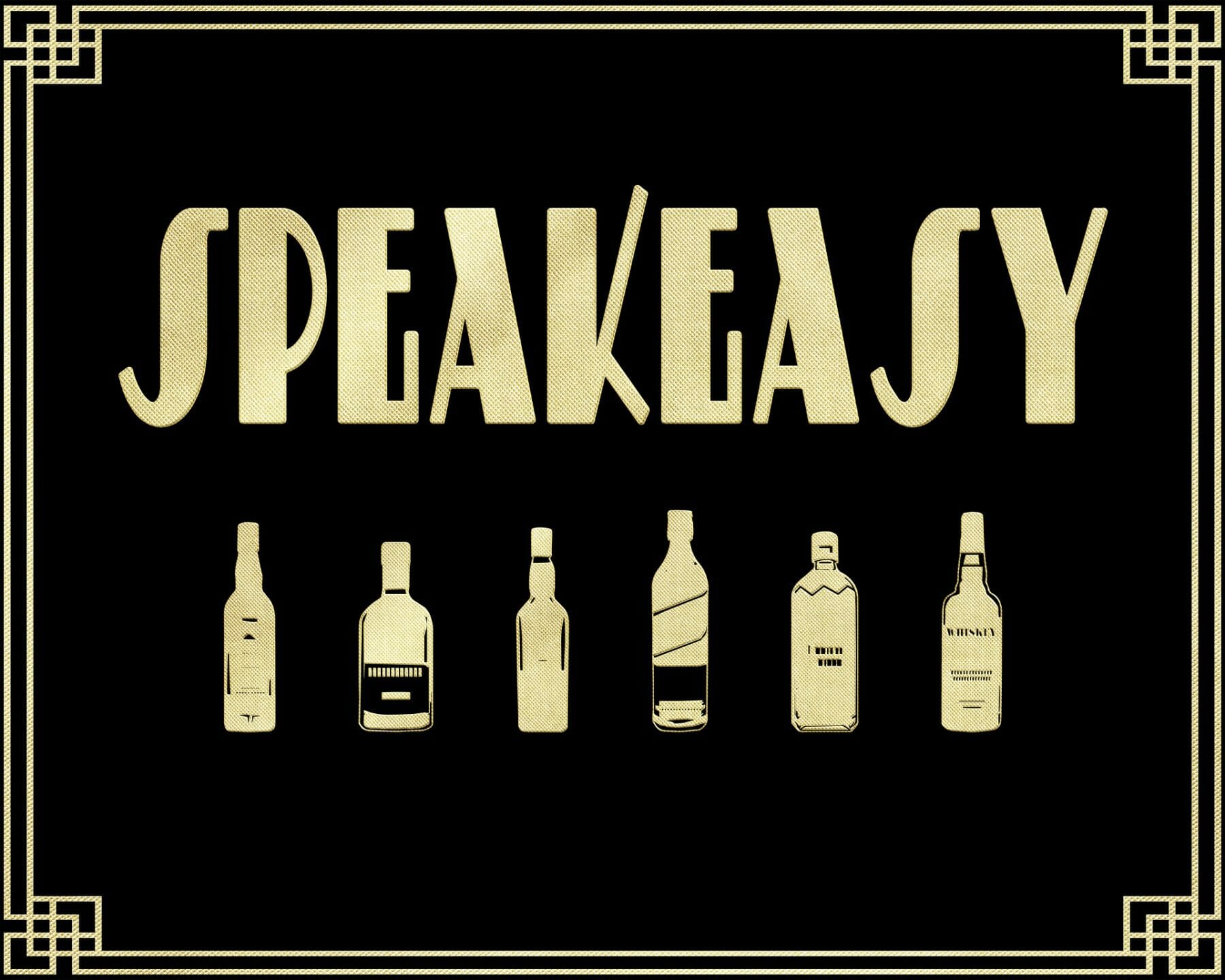This image depicts a highly stylized sign or art piece with a jet black background accentuated by ornate geometric borders in a luxurious gold color. At the top of the design, the word "SPEAKEASY" is prominently displayed in an Art Deco font, written entirely in capital letters. Below this elegant lettering, six distinct liquor bottles, each outlined in the same gold hue, are arrayed. While some of the bottles are identifiable—such as whiskey—others remain ambiguous, representing a mix of gin, scotch, and possibly bourbon. The design is clean and crisp, with the gold elements contrasting sharply against the dark background, rendering a sophisticated, vintage aesthetic reminiscent of an old-time speakeasy bar sign. The border's intricate patterns further enhance the artwork, evoking a sense of refined decadence and nostalgia.